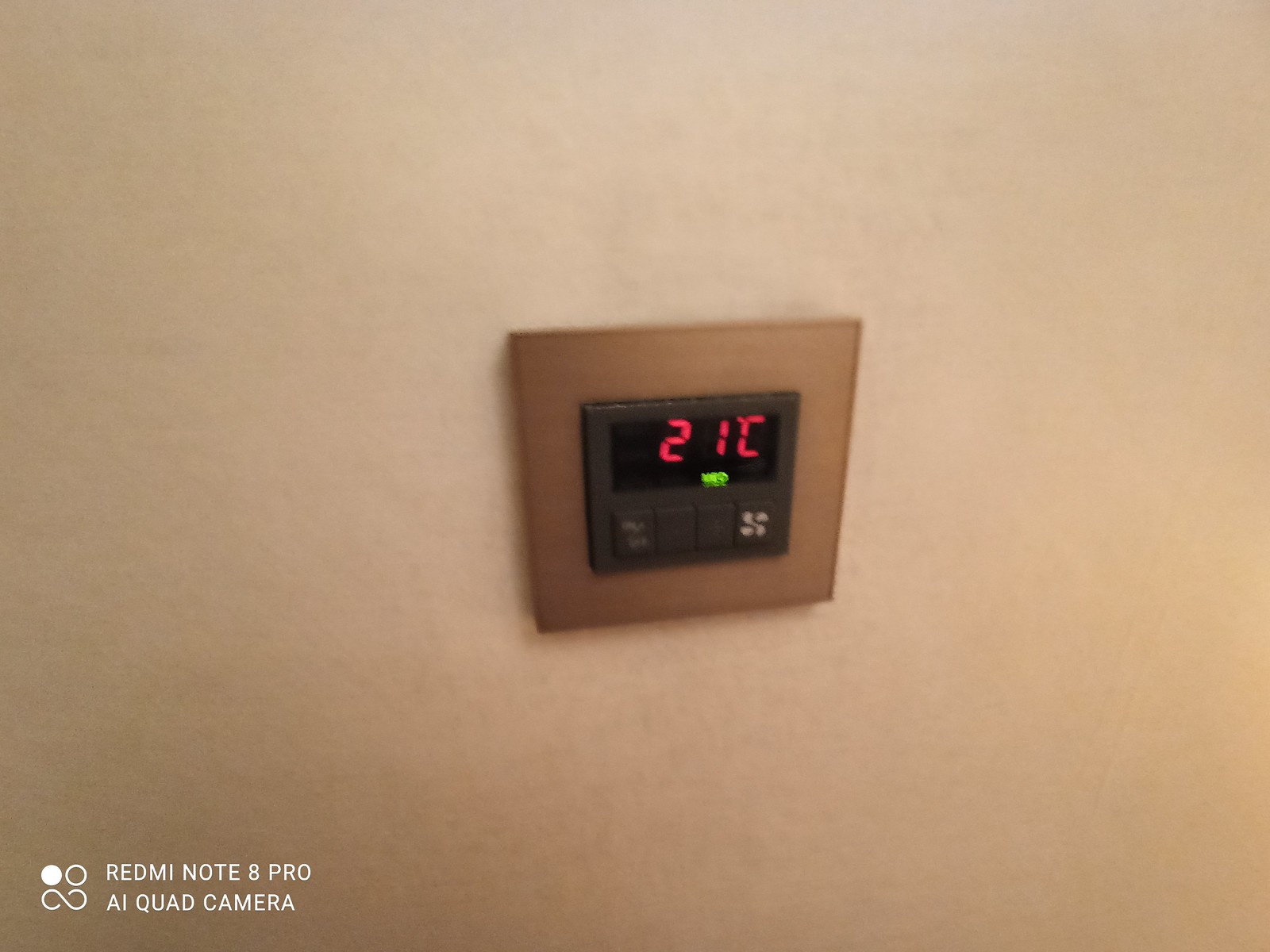The photograph captures a thermostat mounted on a light peach-colored wall. Positioned centrally, the thermostat features a sleek black face encased within a brown square frame. Prominently displayed on the black interface, a red illuminated temperature setting reads 21 degrees Celsius. Below this, faint green neon text appears, though it is too blurry to decipher. The thermostat interface also includes four additional buttons aligned in a row at the bottom, with the last button marked by a fan symbol.